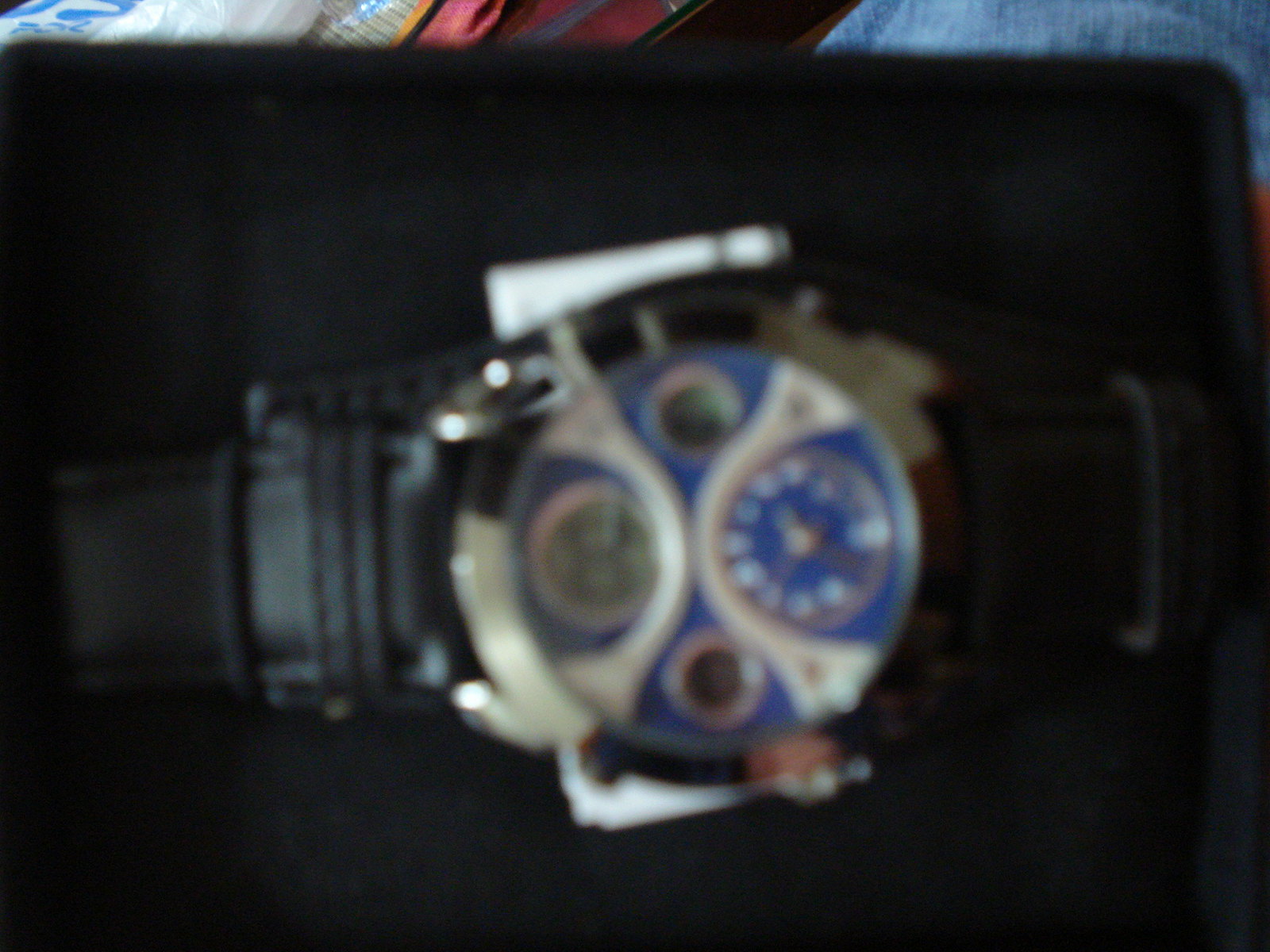This image showcases a watch with a black leather band, though the photo is extremely blurry, making it difficult to distinguish fine details. The watch is positioned horizontally with the band extending to both the right and the left of the frame, and the face centered. The watch face itself is blue and features white accents, along with four smaller sub-dials that are indistinguishable due to the blur. The background of the image is primarily black, but there is a thin, clear strip at the top revealing what appears to be a person’s leg clad in jeans, alongside some red objects, possibly shopping bags. It seems like the close-up attempt to photograph the watch resulted in the distant background being more in focus than the watch itself.